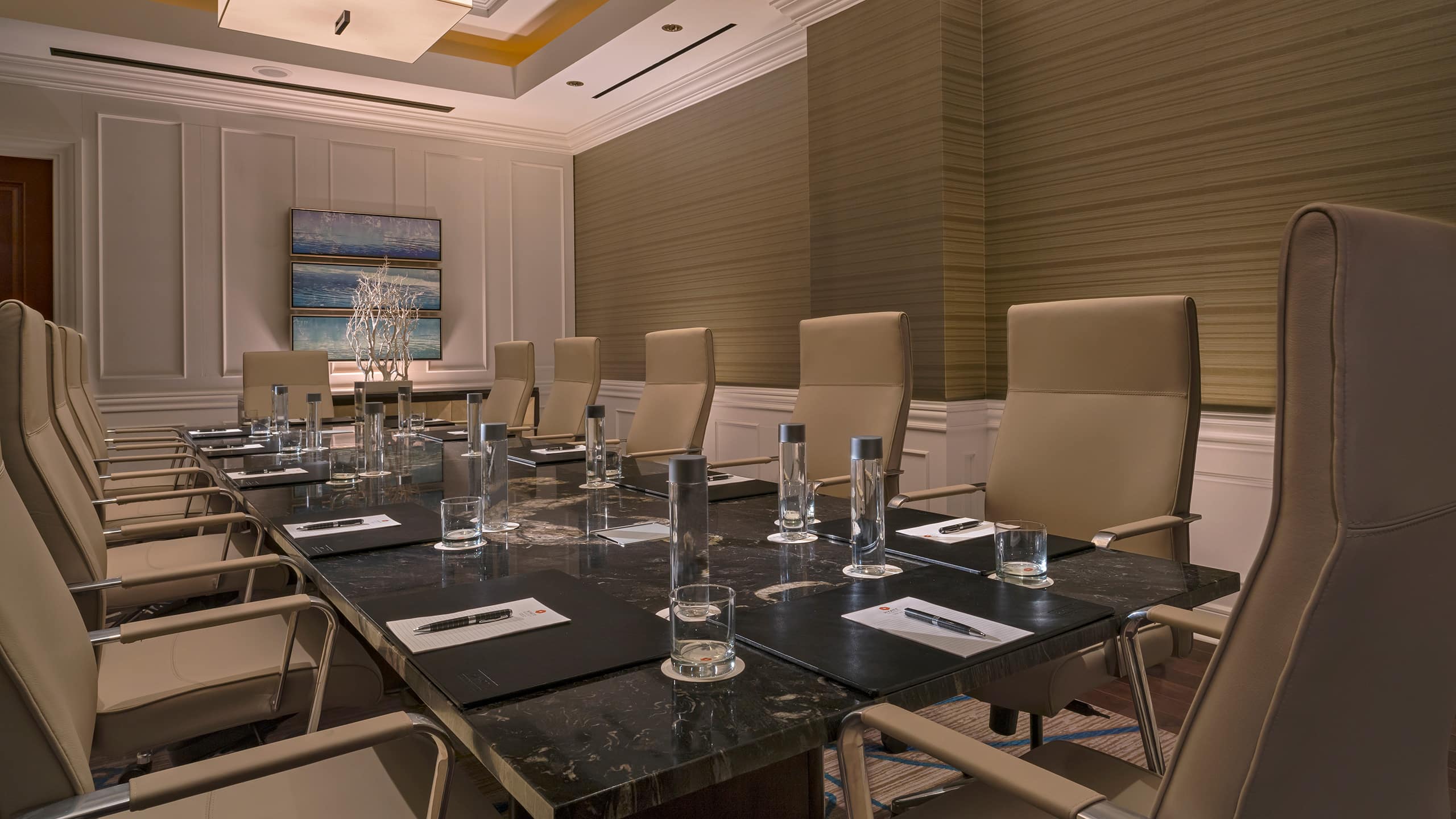This photograph captures a modern, sharply defined conference room. Dominated by a contemporary black marbled table, the room boasts twelve high-backed, tan leather chairs, each featuring matching armrests. The place settings are meticulously arranged: each includes a black leather placemat topped with a white notepad and a pen, anticipating note-taking. A small glass, seated on a coaster, and a sleek, cylindrical bottle of water with a silver top complement each setting. The walls exhibit contrasting styles; one is cream-colored adorned with empty frames and a three-piece vertical scenic artwork, while the other showcases taupe wallpaper with dark horizontal stripes and white wainscoting below. An abstract triptych in shades of blue, teal, and white serves as a focal point. The overall ambiance is one of modern elegance and precision.